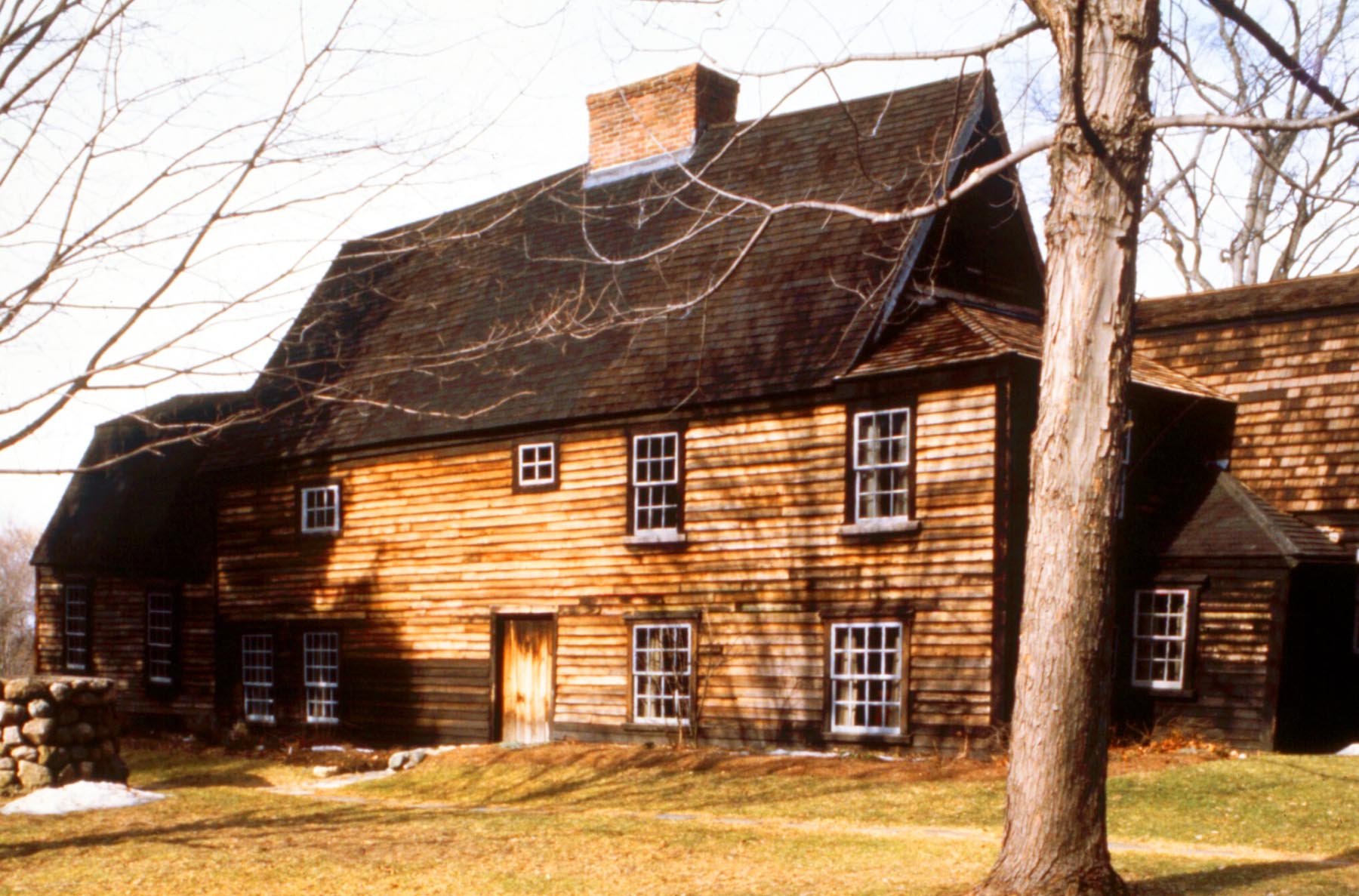The photograph captures the side view of a historical, multi-storied wooden house, likely from the early colonial era, now modernized with new windows. The house, which stands tall under a partly cloudy sky with patches of blue, has a steep, pointed roof with dark brown and black shingles, and features a prominent rectangular brick chimney at its center. The structure includes several compartments with a smaller wing on the left and a shed on the right. The exterior showcases untreated or unpainted wooden planks, giving it a rustic appearance. Despite the old-world charm, it's been updated as indicated by the modern windows with white frames that come in various sizes, with eight visible windows in total—two on the left and one on the right. A plain wooden door is situated on the side. In front of the house is an old, gray stone well, enhancing the historic ambiance. A tall, barren tree stands on the right, and several other leafless trees are scattered around, suggesting it's winter. The brown grass is interspersed with small patches of snow, and a dirt pathway bordered by grass leads to the front door, which is accompanied by a stone step.